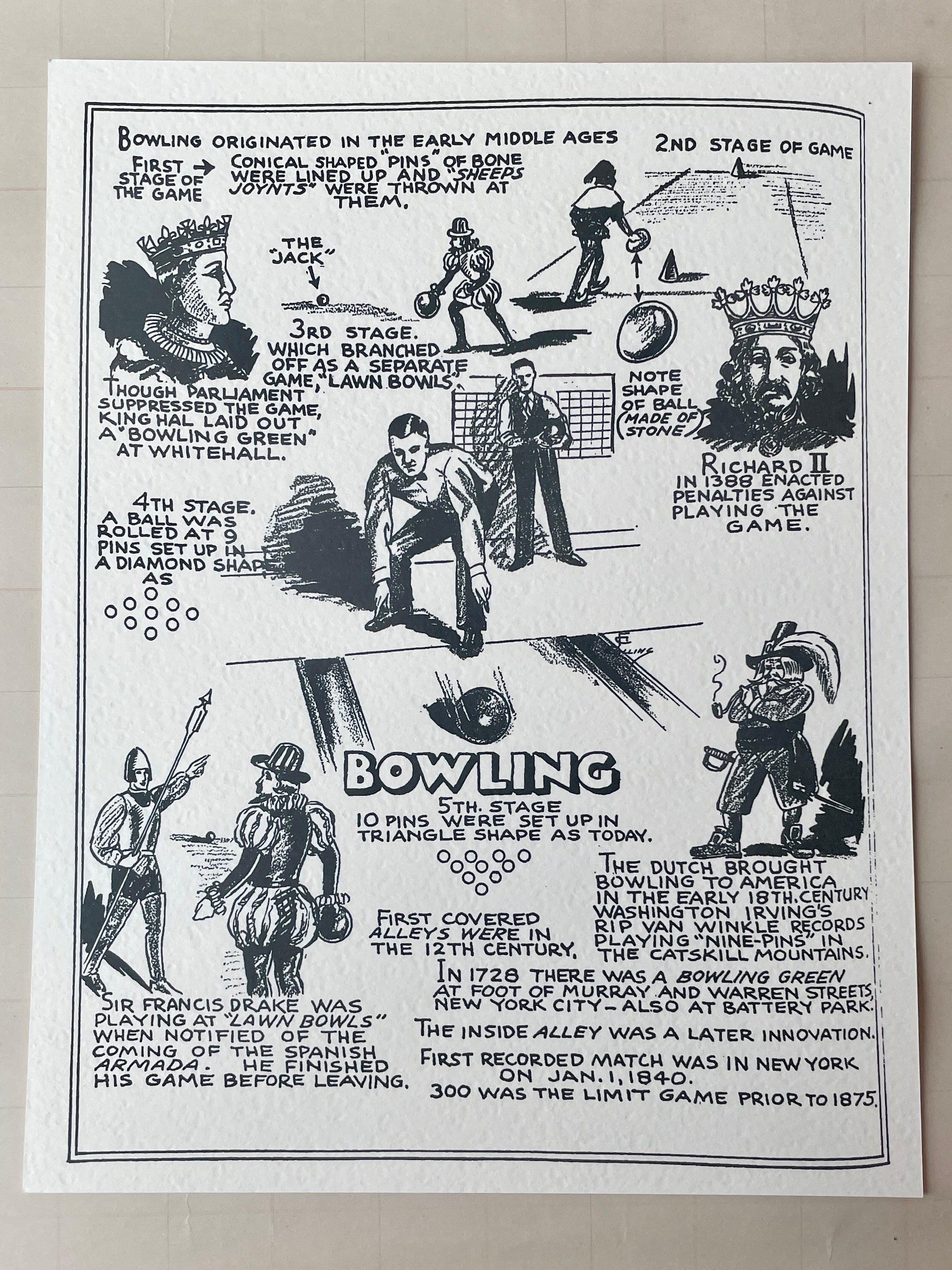The image is a detailed, hand-drawn infographic in black and white, depicting the history and evolution of bowling. The text across the top reads, "Bowling originated in the early Middle Ages." The infographic comprises numerous simple illustrations and handwritten comic-style text. It begins with the first stage, where conical-shaped pins made of bone were set up, and sheep’s joints were thrown at them. It progresses through various stages, showing the transformation from medieval players to Victorian-era individuals. The second stage details the use of stone balls and notes Richard II’s penalties against the game in 1388. The third stage shows the branching off into lawn bowls, mentioning that King Hal established a bowling green at Whitehall. The fourth stage depicts a ball being rolled at nine pins arranged in a diamond shape. Finally, the fifth stage shows the modern ten-pin arrangement in a triangle shape. The infographic also highlights the Dutch influence, bringing bowling to America in the early 18th century, and mentions Washington Irving's description of playing nine pins in the Catskill Mountains. It notes a bowling green established in 1728 at the foot of Murray and Warren streets in New York City. The hand-drawn images and text create a visually engaging and educational depiction of bowling’s storied past.